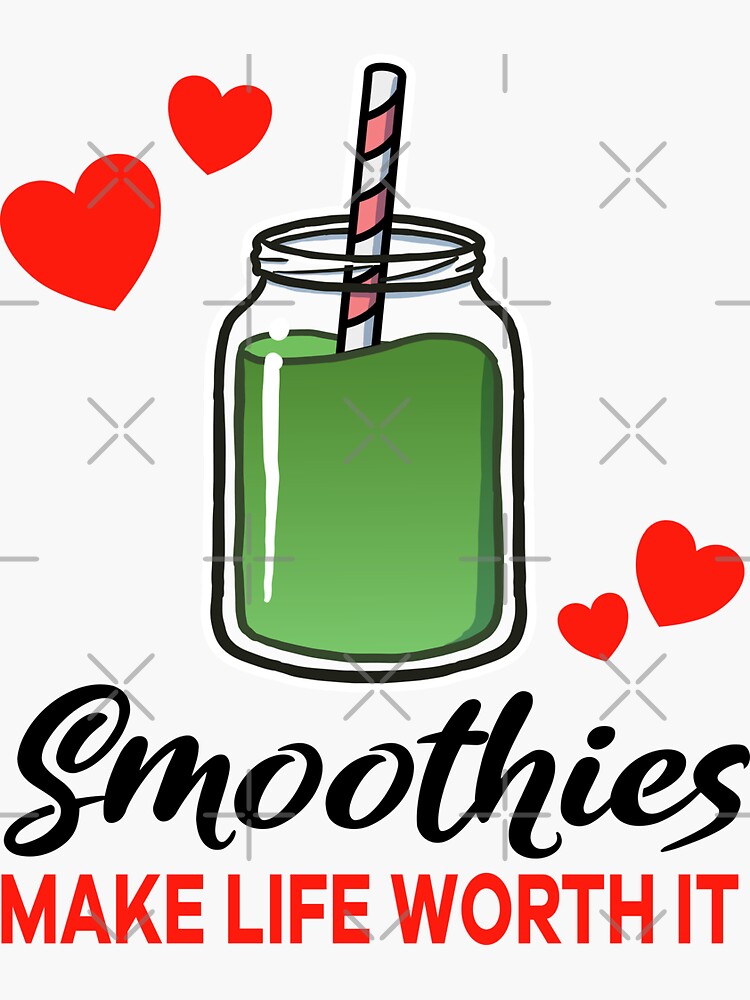This is a playful and whimsical illustration of an advertisement for "Smitty's Smoothies," featuring the tagline "Make Life Worth It." The image is in a rectangular format with a light gray background adorned with alternating rows of gray X's and dashes. Scattered throughout are various red hearts, which add a charming touch to the design.

At the center of the illustration, a jar filled with a green smoothie is prominently displayed. The jar is drawn with thick, bold lines and has a pink and white striped straw standing vertically in the middle. The green liquid inside the jar gradates from a darker shade at the top to a lighter shade at the bottom, and a highlight accents the left side of the jar. The whimsical character of the illustration is heightened by the playful elements floating around the jar, including the hearts.

At the bottom of the image, "Smitty's" is written in black script font, while "Make Life Worth It" is boldly displayed in vivid red letters. The overall aesthetic of the illustration is cartoonish and fun, making it both visually engaging and inviting.